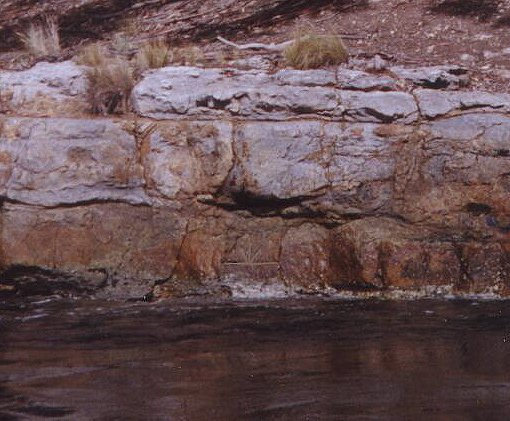The photograph captures a serene and natural scene featuring a rock wall adjacent to a body of water. The image has a slight rectangular shape, with the top and bottom edges marginally longer than the sides. Occupying the bottom one-third of the frame, the water appears dark gray and flows gently from left to right. Its reflective surface mirrors the surrounding environment, adding depth to the scene.

Dominating the rest of the photograph is a large, tiered rock wall. The base of the wall is brown and damp, seamlessly transitioning to a mix of gray and white in its middle and upper sections. Patches of brown intersperse the middle section, while the top is predominantly white with small clusters of gray and green grass sprouting from it.

Beyond the rock wall, a sloped expanse of brown soil is visible. This area is speckled with white rocks and dotted with dried vegetation, tracing an upward path out of the frame. The intricate textures and earthy tones create a harmonious blend between the rock formation and the surrounding landscape, evoking a sense of untouched natural beauty.